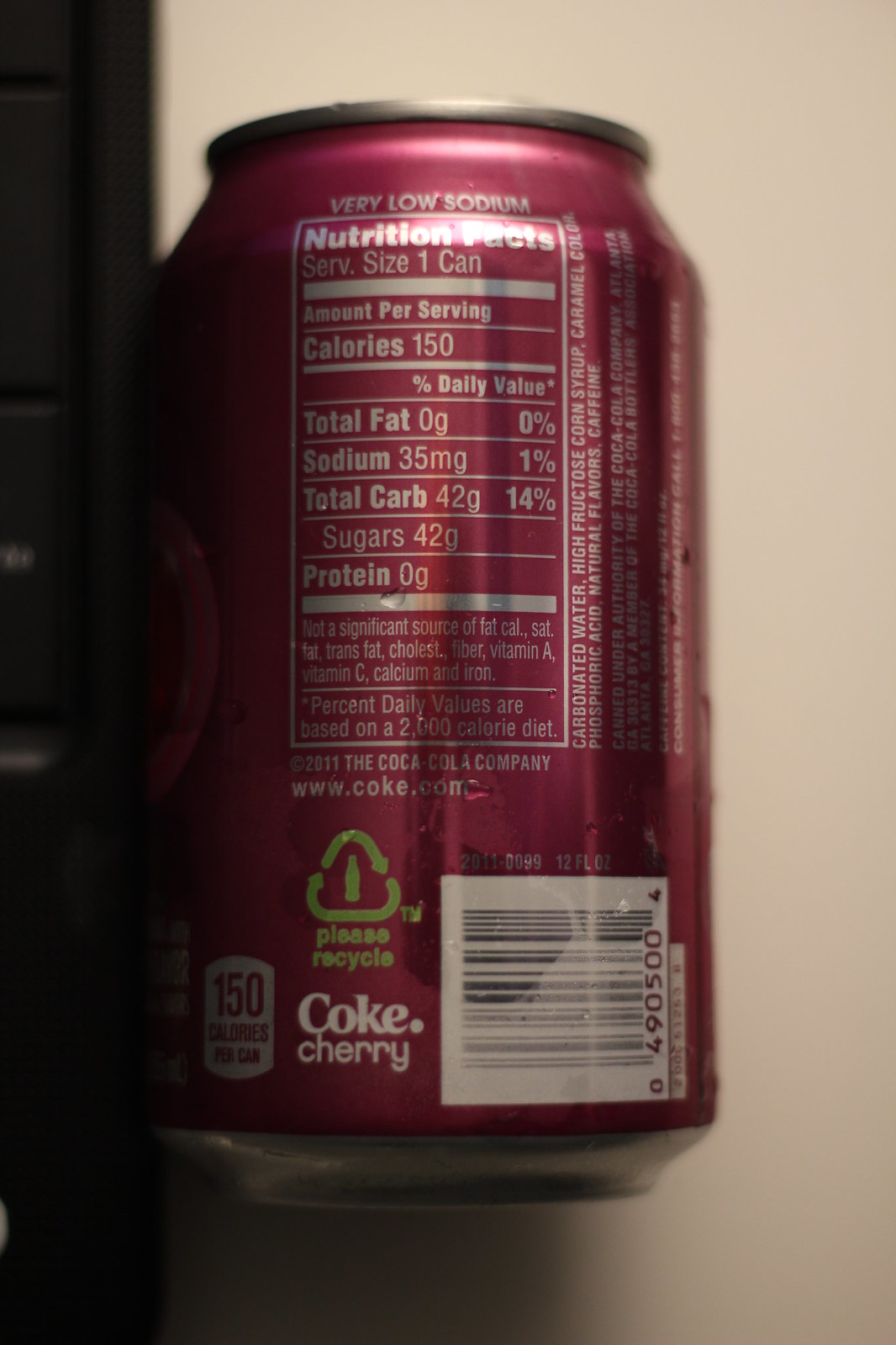This close-up photo captures the back of a Coca-Cola can against a background divided into a tan area on the right and a vertical black strip along the left edge. The can itself is prominently centered in the frame. The top of the can is silver, while the rest of the background is a vivid red. Noticeably, the nutritional facts box near the top is outlined and detailed in silver, presenting all nutritional information in the same hue. Beneath this box, there are two lines of white text. Further down, a distinctive lime green triangle with rounded edges is visible, featuring a thick green vertical line down its center. Below this triangle are two rows, each containing a single word. Continuing downward, the word "Coke" appears in white, followed by "cherry" directly beneath it. Adjacent to the word "cherry," on the right, lies the white square designated for the UPC code.